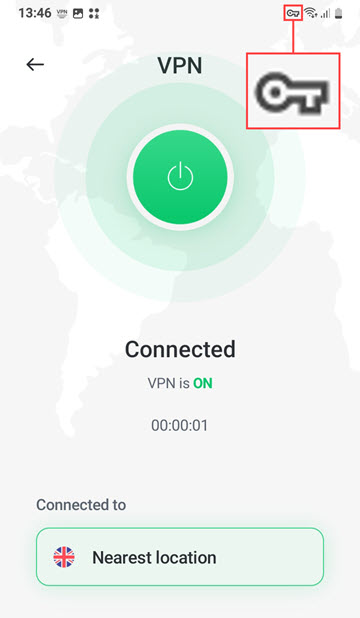This image is a screenshot from an Android mobile device, as indicated by the gray, bold text in the top left corner displaying the time "13:46." There are three icons to the right of the time: the first icon is unidentifiable, the second is an image icon, and the third consists of four dots forming a square. Towards the far right, there is a small gray key icon outlined by a red square with a red line extending downwards. Below this, a magnified version of the key icon is displayed within a larger red square border.

On the left side of the screen, there is a gray left-arrow icon. At the center, the text "VPN" is prominently displayed in capital letters. Below this, a lime green icon with a light green or white power symbol is enclosed within a white circular border. Surrounding the white border is a semi-transparent, light green circular area followed by a light gray circular border. The "VPN" text is situated within this gray border.

Beneath this central visual element, the word "connected" appears in black text. The background features a gray and white map of the continents. Directly underneath the word "connected," the text "VPN IS ON" is displayed, with "VPN" in gray capital letters, "is" in gray lowercase, and "ON" in bold lime green capital letters. Below this, a timer reads "00:00:01" in gray font. Finally, at the bottom left, the text "connected to" appears in gray.